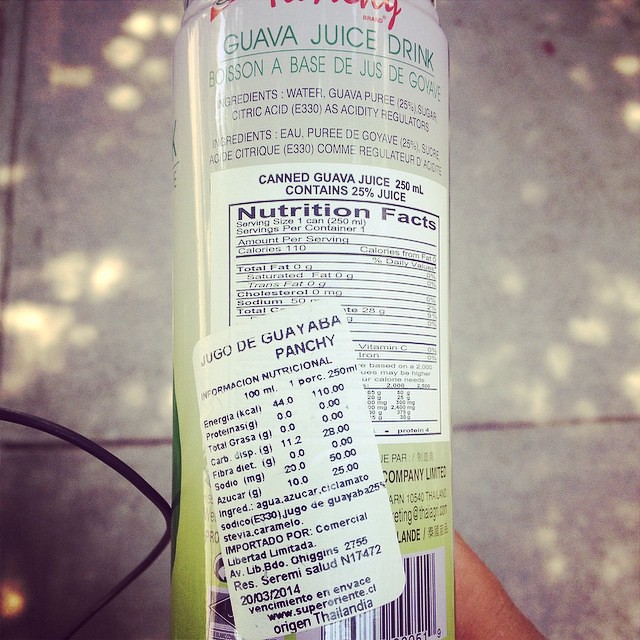In this color photograph taken outdoors against a sidewalk background, a hand holds a tall, slender can of guava juice drink, viewed from the back. The can's top is a silver-white color with green text reading "Guava Juice Drink." Below this, a bilingual section includes ingredients listed as "Water, Guava Puree (25%), Sugar, Citric Acid, Acidity Regulators," followed by the ingredients in another language. Next is a white label with black text displaying "Canned Guava Juice, 250 ml, Contains 25% Juice," along with a detailed table of nutritional facts. A white sticker partially covers this section, featuring text in another language, possibly Spanish, indicating "Jogo, The Guava Punch," and a website link, highlighting its Thai origin and a barcode at the bottom. The bottom-right corner of the image shows the tip of the lightly tanned finger holding the can.